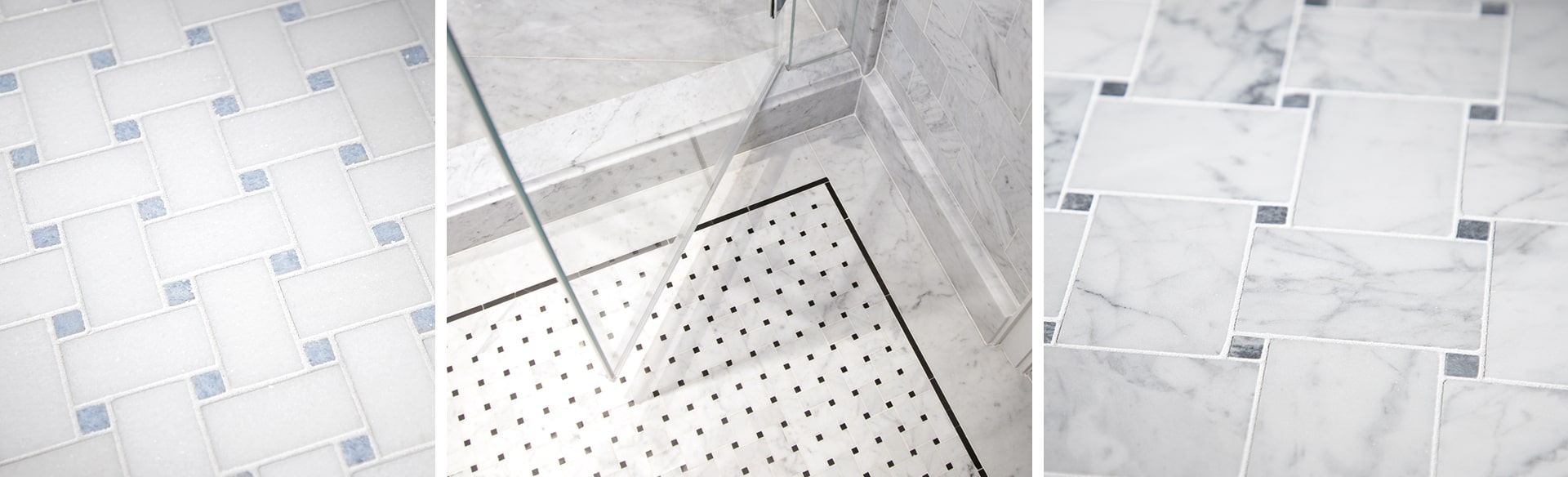This image consists of three distinct photographs showcasing various types of bathroom flooring. The first photograph on the left features a basket weave pattern with white lines interwoven on a blue-gray background, creating a striking contrast. The middle photograph captures the interior of a modern shower, where the walls are adorned with white and gray marble. The shower floor boasts a white background with black polka dots, bordered by a black outline, and a glass door stands ajar. The third photograph on the right depicts a closer view of another basket weave pattern, similar to the first, but here the interwoven lines are a white and gray granite against a dark gray granite background. Each photo offers a unique and detailed perspective on stylish bathroom flooring options.